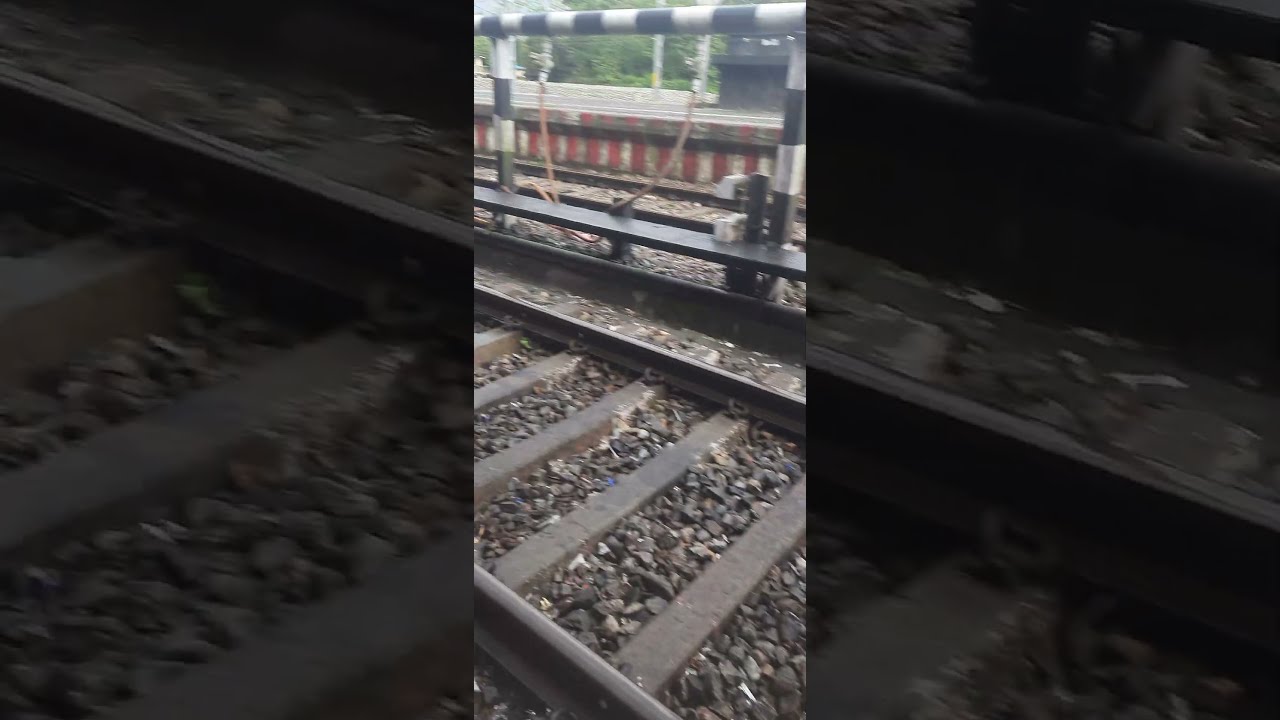This daytime photograph captures a segment of railroad tracks, likely situated at a train station. The image features a pair of steel rails running diagonally from the lower right to the mid-center of the frame, intersected by wooden planks and surrounded by dark gravel stones. A notable element is a black and white striped barrier, accompanied by rope, suggesting a crossing or safety feature. Beyond the tracks, a concrete platform is visible, marked with red vertical stripes and some benches or seats. The background shows distant trees and additional station infrastructure, reinforcing the setting's train station ambiance.